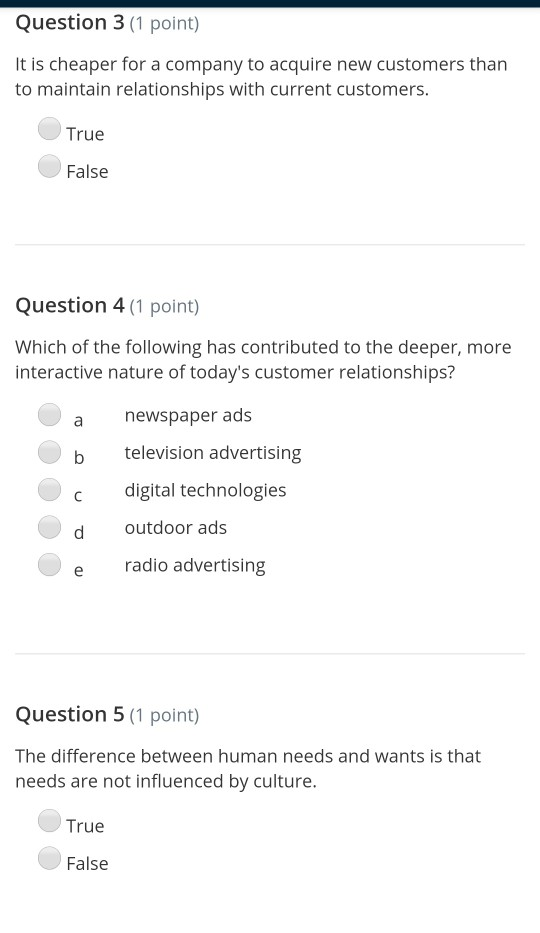The image displays an online test on customer relationships and marketing strategies. At the top, there's a thin black bar spanning from the left to the right. Below this, on the left, it reads "Question 3" followed by "(1 point)" in gray. The question states, "It is cheaper for a company to acquire new customers rather than maintain relationships with current customers," with two options below: a white circle labeled "True" and another labeled "False."

Following this, a light gray bar appears before "Question 4 (1 point)" is presented in the same format. The question asks, "Which of the following has contributed to the deeper, more interactive nature of today's customer relationships?" with five options labeled A through E. The choices listed are:
- A: Newspaper Ads
- B: Television Advertising
- C: Digital Technologies
- D: Outdoor Ads
- E: Radio Advertising

Another gray bar demarcates the end of question four and leads into "Question 5 (1 point)." This question inquires about the difference between human needs and wants, stating, "Needs are not influenced by culture," with similar options: "True" and "False."

The test appears to be nearing completion, with just a few seconds left for submission.